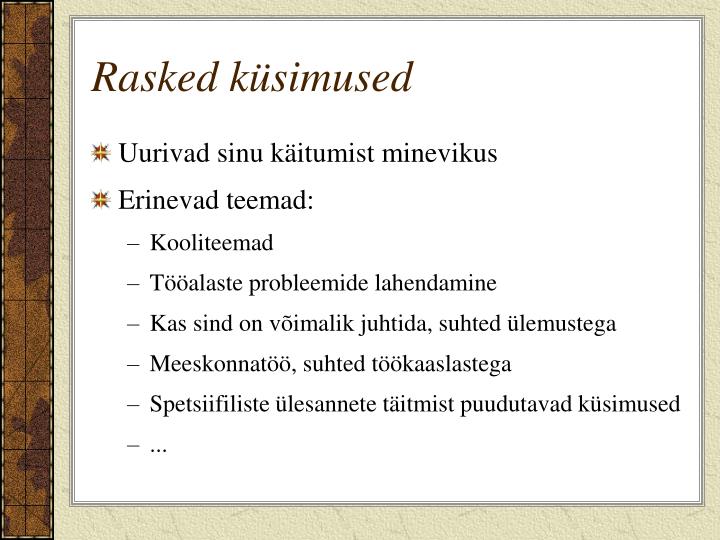The image shows a PowerPoint slide with a title in a non-English language that might be Germanic or Nordic, reading "Rasked Kusumused." The slide has a decorative vertical stripe on the left side, colored in shades of brown, resembling an old map. The background has a parchment-like texture, while the text is placed within a plain white textbox that almost completely covers the slide. The text within the textbox is in black, featuring several bullet points. The first bullet point stands alone with no sub-points, while the second bullet point has a colon after it and is followed by five sub-points. At the end of the list, there is a sixth bullet point marked with ellipses, indicating continuation.